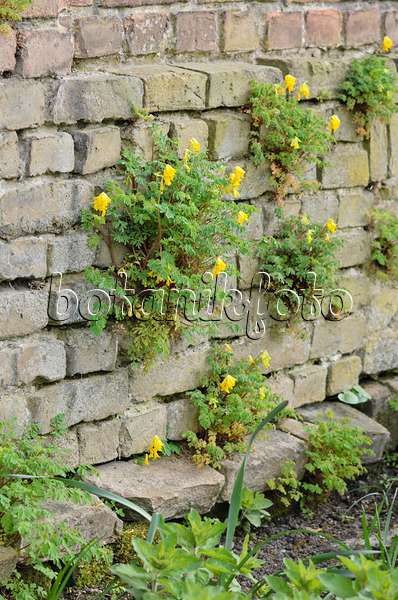This color photograph captures a section of a very old, brown and light tan brick wall, characterized by noticeable creases between each brick. The wall is partially surrounded and interspersed with various green shrubs, some of which bear bright yellow flowers that frequently punctuate the scene. In front of the wall, there is a dirt area where additional green leafy plants, distinct from those growing through the wall, can be seen. Centered across the image, a translucent watermark spells out "B-O-T-A-N-I-K-F-O-T-O." The image is void of any people or animals and depicts an idyllic, possibly garden-like setting.